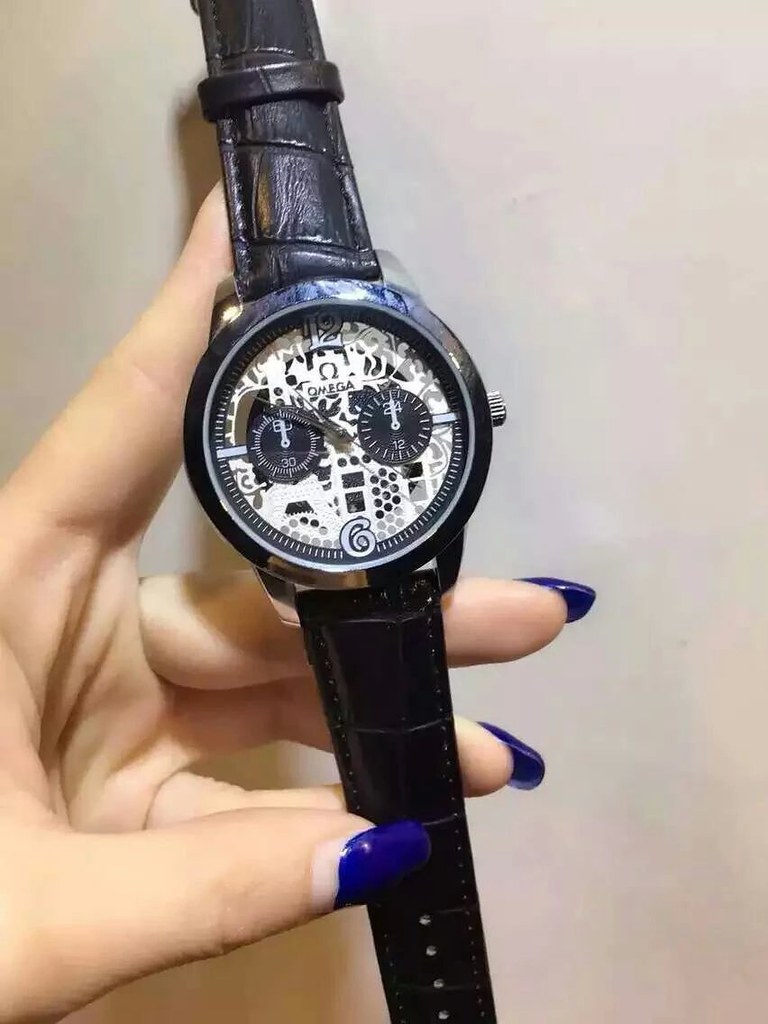This detailed photograph captures an elegant Omega wristwatch being gracefully held by a woman's left hand, adorned with long blue nails, predominantly blue at the tips. The white or light gray background serves to highlight the intricate details of the watch. The Omega watch features a black leather band with a croco design, segmented with tiny punched holes along the outer lengths. The silver-toned watch has a white clock face, meticulously designed to showcase only the 12 and 6 numerals, positioned at the top and bottom, respectively.

The watch face includes additional complications: on the right side, a 24-hour clock, and on the left, a second counter marked with a “30” at the bottom. The watch hands are exceptionally thin, dark gray metallic lines without pointed arrows. The Omega logo and dark gray (nearly black) writing are prominently displayed on the white clock face, adding to the timepiece's ornate and impressive design. The woman holds the watch carefully, with her thumb and fingers supporting it, presenting a clear view of this sophisticated and detailed timepiece against the minimalist background.